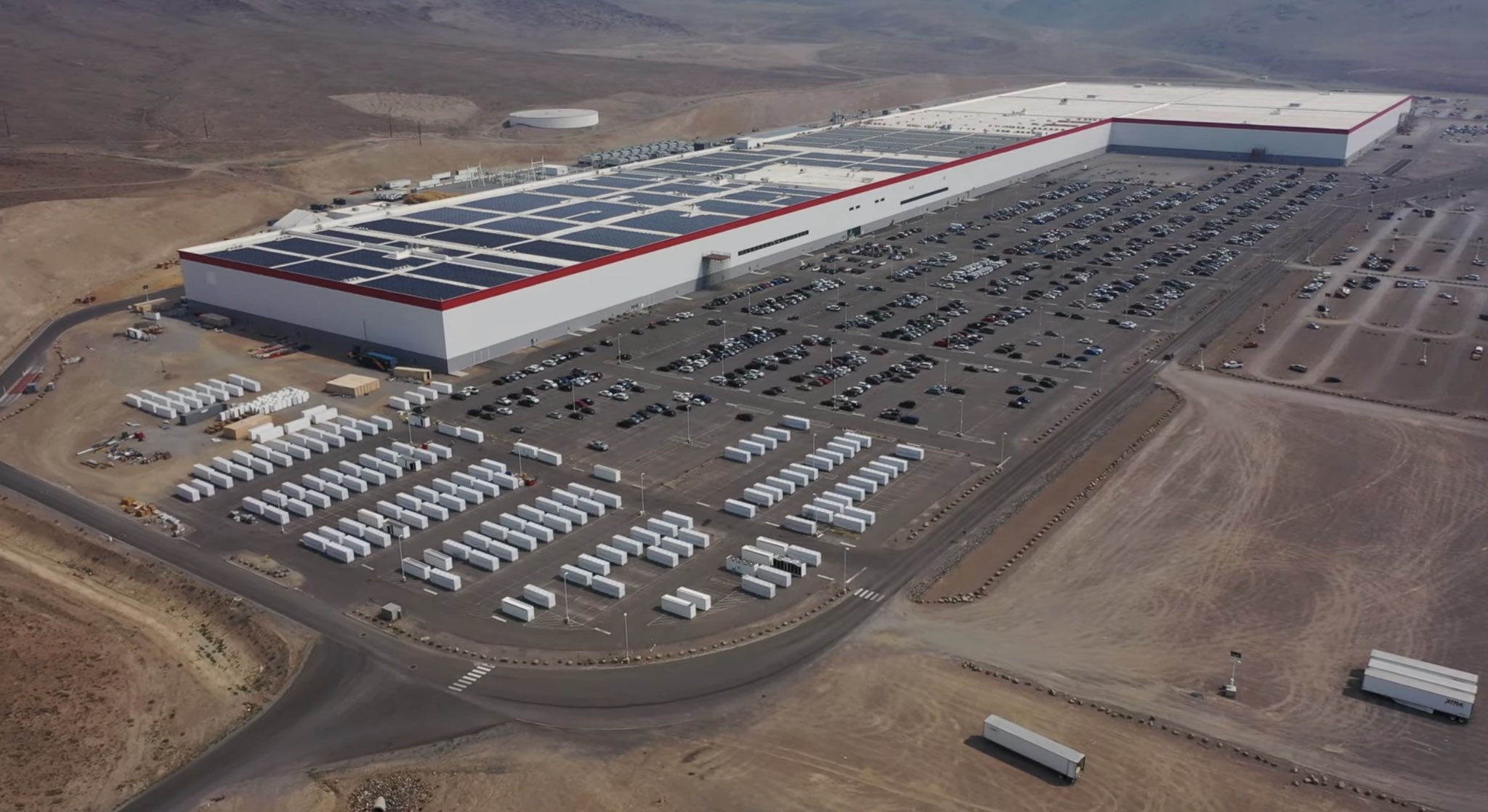The image depicts a vast industrial warehouse or factory, captured from an overhead angle. The main building, predominantly white with a red stripe around the top and a gray stripe at the base, is rectangular and expansive, stretching almost the entire length of the image before forming an L-shape with an adjoining structure. Although the building appears short, standing at one to two stories tall, its footprint is immense, comparable to the size of a shopping mall or three football fields.

Surrounding the building is a large, barren area undergoing development, with plowed and leveled land indicating future construction. The landscape is mostly devoid of grass and trees, giving a dusty, desert-like appearance. Adjacent to the warehouse is an enormous parking lot, densely packed with cars and commercial truck trailers. Scattered around the premises are numerous storage containers, boxes, and pallets, implying active industrial operations.

In addition to ground activities, a water tank is also visible on the property, and there is a suggestion that solar panels may be installed on the rooftop to harness energy. The presence of small doors around the structure, with a door aligning with the gray base stripe, suggests the possibility of a loading dock on the obscured side of the building. The image captures the scale and operational complexity of this industrial site vividly.